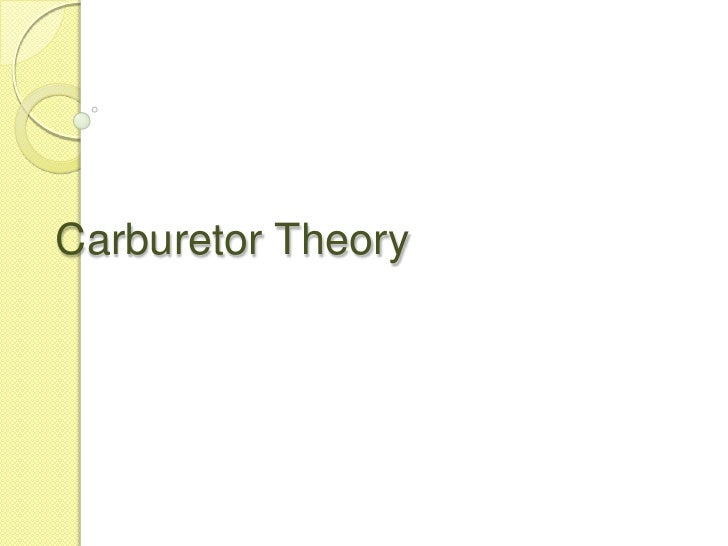The minimalist PowerPoint slide features a predominantly white background with a decorative yellowish-beige vertical strip on the left side. This strip includes a half-circle arc at the top, a smaller, nearly full circle below it, and a few small bubbles. Centered on the slide, overlapping slightly with the yellow strip, are the words "Carburetor Theory" written in a dark green sans-serif font with a faint shadow effect. The capital "C" of "Carburetor" encroaches on the decorative strip, while the rest of the text remains in the white space, creating an overall balanced yet simple design.